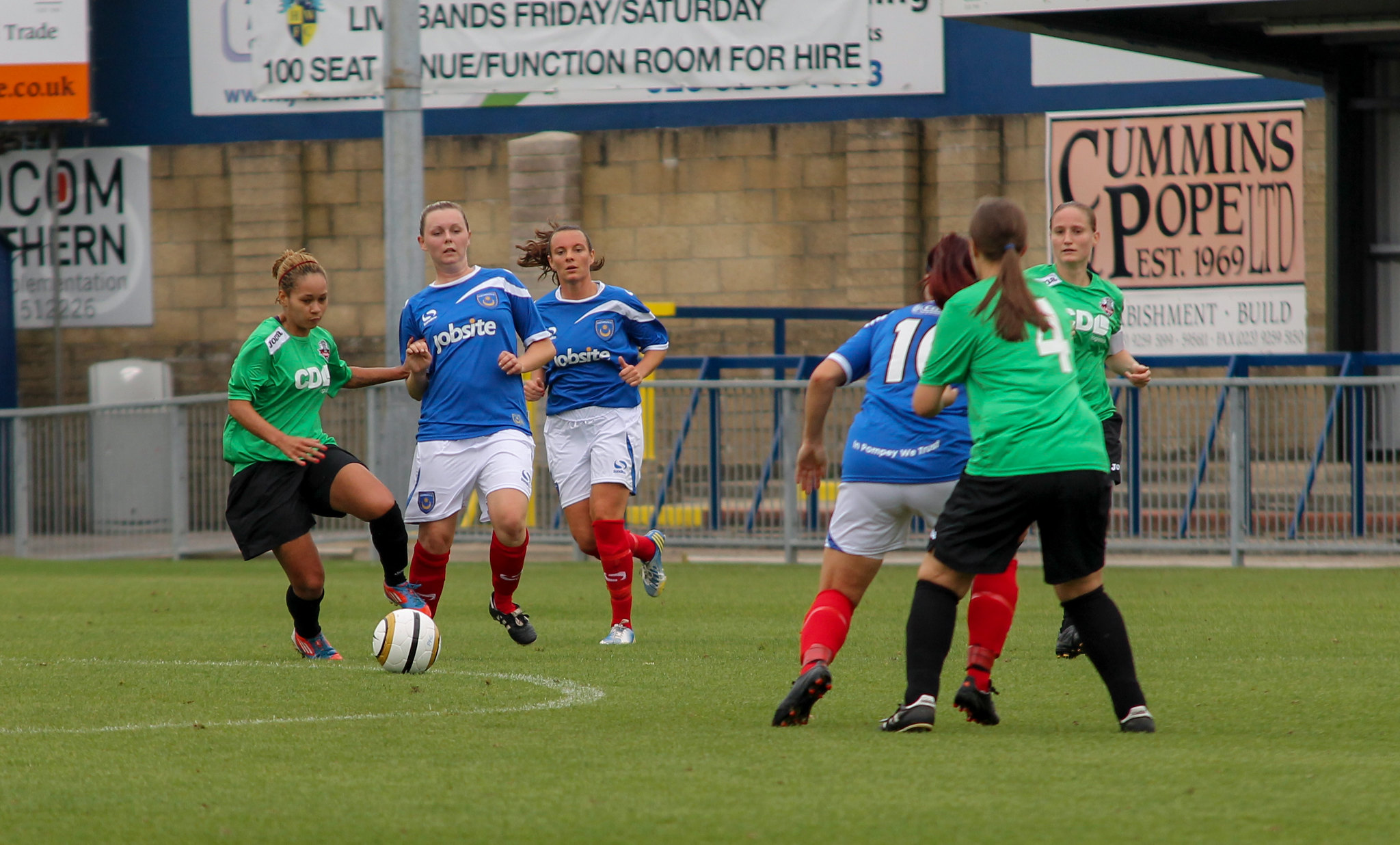This detailed color photograph captures a women's soccer match on a lush green field, framed in landscape orientation. At the heart of the action, six female players are the focal point: three in green jerseys with black shorts and black socks, and three in blue jerseys with white shorts and red socks. The players in blue have "Job Site" emblazoned in white on the front of their jerseys. Among the green team, the player on the far right has the number four on her back. Most players are converging towards a ball located left-center in the image, their attention firmly fixed on it.

In the background, a gray concrete block wall is adorned with several sponsor signs. One prominent sign reads "Cummins Pope LTD EST 1969 Bishman Building," while another partially obstructed sign states "Live Bands Friday-Saturday 100 seat function room for hire." A grey metal fence surrounds the pitch, adding to the enclosed sporting atmosphere. Additional signage is present but partially cut off, only revealing the word "trade." The image, rich in details, showcases a mix of athletic intensity and the everyday elements of a community sports venue, captured in sharp, realistic detail.